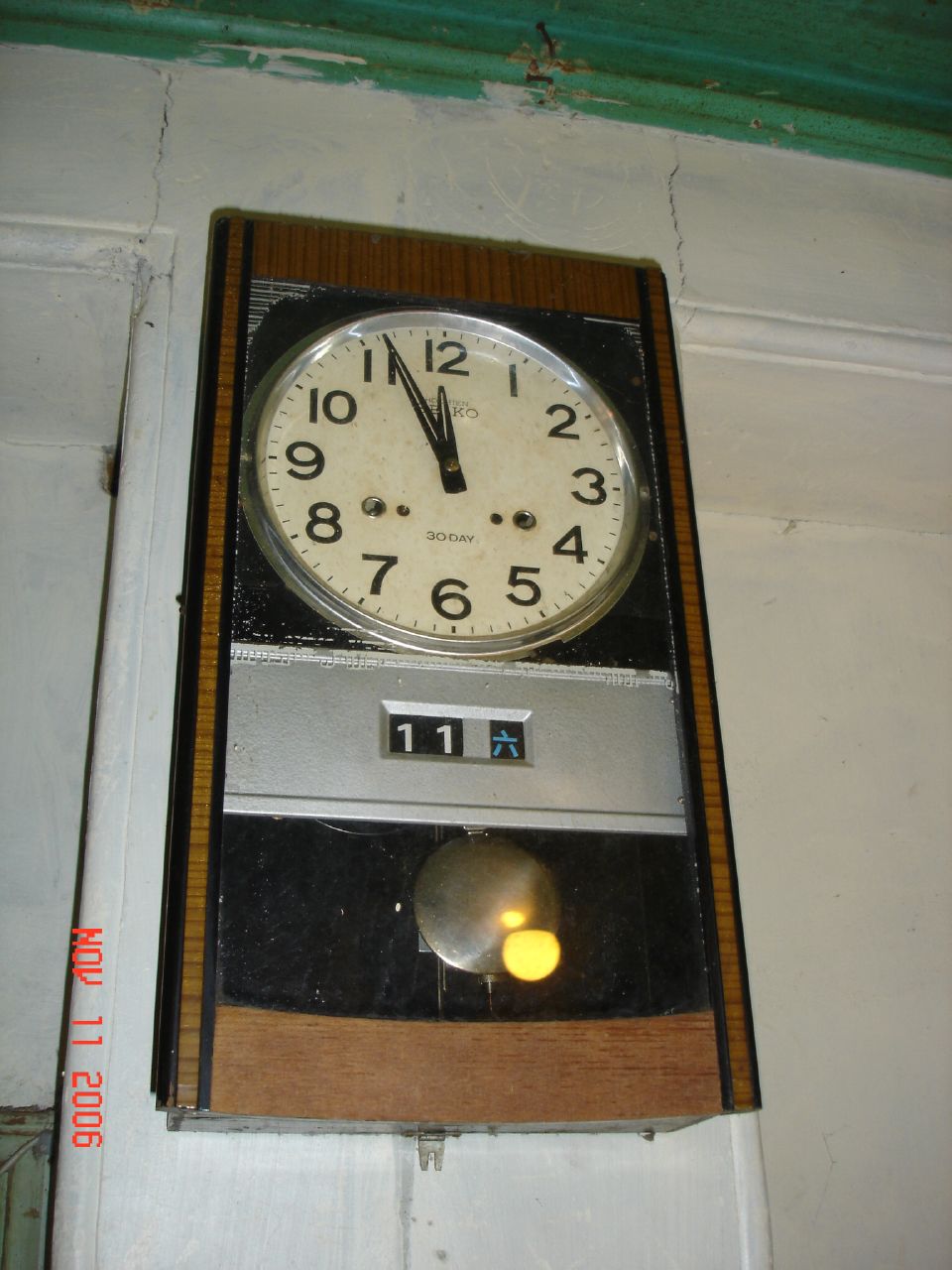This image, captured with a digital camera on November 11, 2006, features a wall-mounted clock as its centerpiece. The timestamp in red lettering is located vertically in the bottom left corner. The wall is white but visibly aged, showcasing a few cracks and thin paint that allows a darker color to subtly show through. At the top of the wall, the green-painted molding frames the scene. The clock is mounted on a wooden panel, with a standard white clock face and black numerals occupying the upper half. The clock shows a time of around 11:56. Below the clock face, a silver band displays the number "11" along with a blue Asian character. Beneath this band, a pendulum swings, completing the elegant yet weathered look of the timepiece.